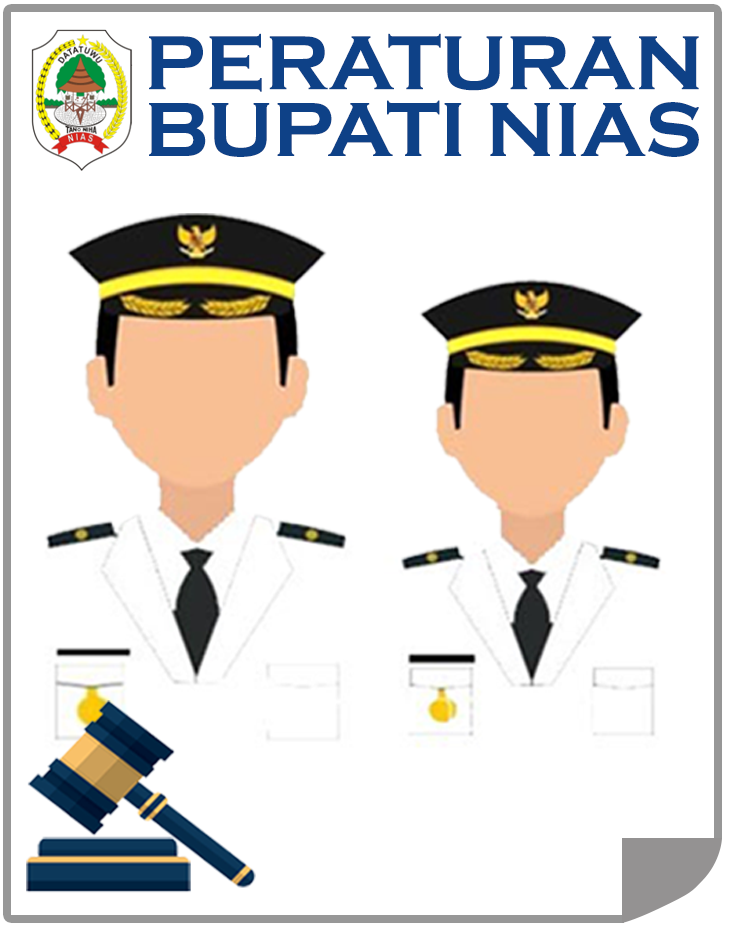This cartoon image is an advertisement or sign with text in a foreign language across the top, reading "Peraturan Bupati Nias" in bold blue capital letters. On the upper left corner, there is a logo or seal featuring yellow stars, a red ribbon, a green tree, and a small brown hut. Below the text, there are caricature-like drawings of two faceless police officers or military personnel, both wearing black hats with a yellow stripe and a gold eagle emblem. They are dressed in white uniforms with black shoulder patches, a black tie, and a gold badge on the right pocket. Notably, their faces are completely blank, lacking any features. In the lower section of the image, there is a navy blue and brown gavel, suggesting a legal or official context.